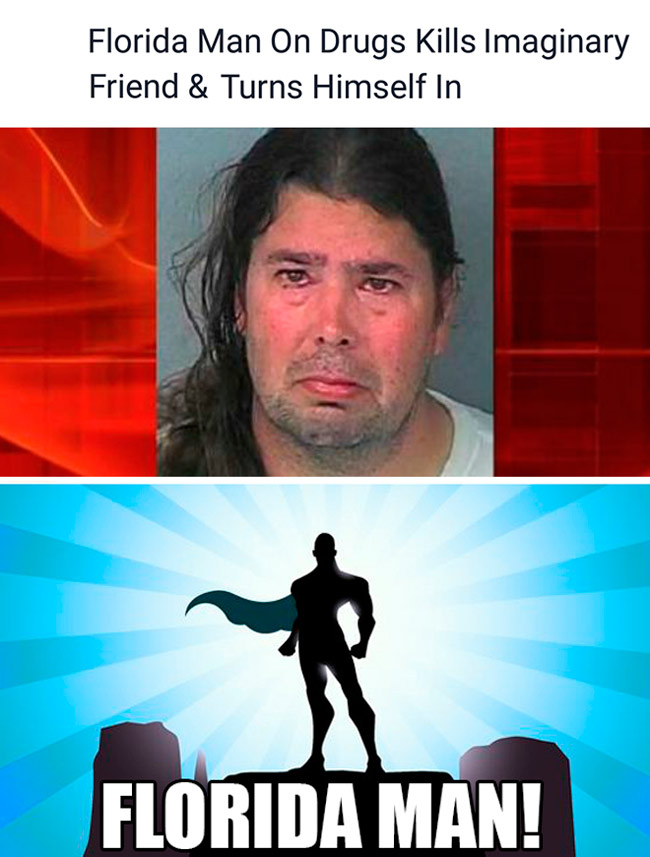The image, structured as a meme, consists of a juxtaposition of two distinct rectangular pictures with descriptive text. At the top, against a white background, bold black text reads, "Florida man on drugs kills imaginary friend and turns himself in." Below this, the upper half of the image features a distressed, overweight white man with long, dark hair and stubble, appearing on the verge of tears and dressed in a white t-shirt. The backdrop includes both a gray color and vertical red bars beside his head, emphasizing his disheveled state. In the lower half, a black silhouette of a superhero with a cape stands triumphantly on a rock-like structure against a blue, sunburst background. Below this silhouette, bold white text declares, "Florida Man!" The contrast between the man's sorrowful mugshot and the superhero caricature satirizes the outlandish headline, emphasizing the stereotype of bizarre news stories emerging from Florida.